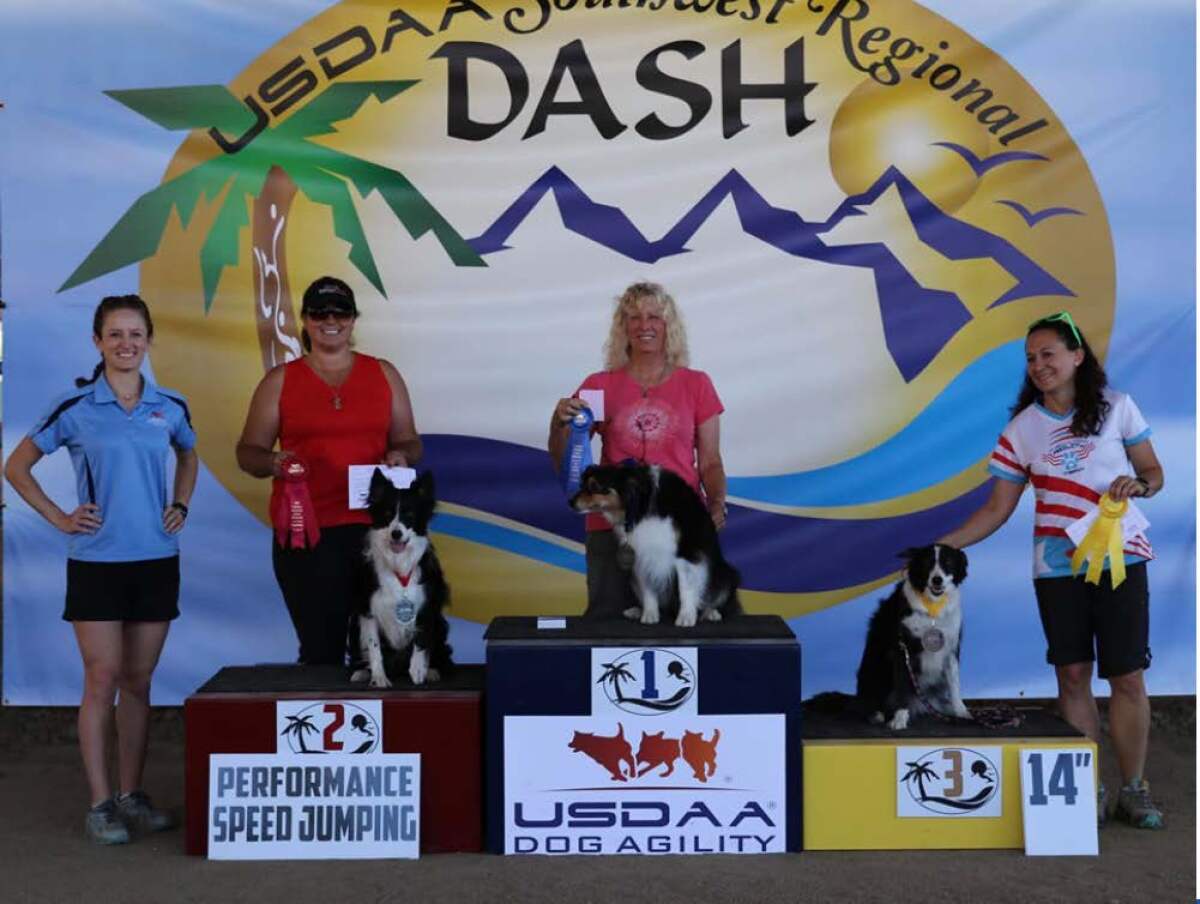This photograph captures the winners of a dog agility test, showcasing a vibrant and celebratory scene. Centrally featured are three black and white dogs standing proudly on podiums labeled with numbers one, two, and three. The middle box, being the highest, signifies the first-place winner, with the second-place box to the left and the third-place box, slightly shorter, to the right. Each dog displays a white chest, with contrasting darker fur predominantly black or brown, distributed over their faces, ears, and bodies.

Four women stand behind the dogs, all dressed in casual clothing like t-shirts, shorts, or yoga pants. Three of these women are holding ribbons: the central woman sports a blue ribbon, indicating first place, while the others proudly hold red and gold ribbons. A fourth person, possibly a judge, stands to the left, distinguishably dressed in a blue shirt.

In the background, an eye-catching banner reads "USDA Southwest Regional Dash," featuring a circular design with illustrations of a palm tree, mountain range, sun, birds, and ocean-like blue swirls. The dogs, especially the first and second place winners, gaze directly at the camera, exuding a sense of achievement and pride. The celebratory and competitive atmosphere is further emphasized by the descriptive signs on the podiums such as “USDA dog agility," “performance speed jumping,” and “14 inches,” hinting at the jumping heights these agile dogs have conquered.